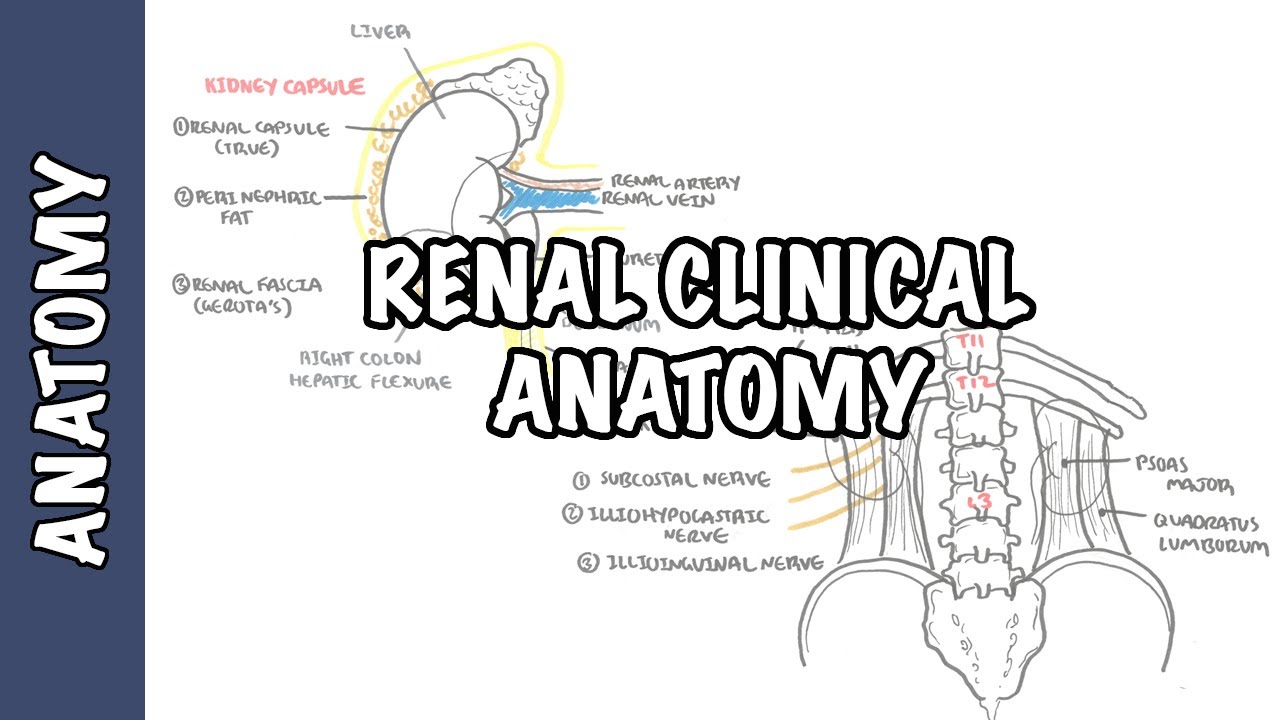The image is a detailed diagram of renal clinical anatomy. On the left side, there's a vertical dark navy blue rectangle with the word "Anatomy" written in white text. Superimposed across the middle of the image in white text are the words "Renal Clinical Anatomy." The central diagram focuses on the renal area, showcasing the kidney, renal capsule, and kidney capsule. It includes directional arrows pointing to various anatomical parts such as the renal fascia, perinephric fat, renal artery, and renal vein. Additional details include portions of the liver and the right colon (hepatic flexure). The labels are enhanced with colors like yellow, red, and brown for better differentiation. In the lower right-hand corner, there's another detailed illustration of the spinal column, hip bones, and associated muscles, clearly labeled with terms like subcostal nerve, iliohypogastric nerve, psoas major, and quadratus lumborum. This composite diagram serves as a comprehensive guide to renal anatomy, highlighting essential structures and their interrelations.